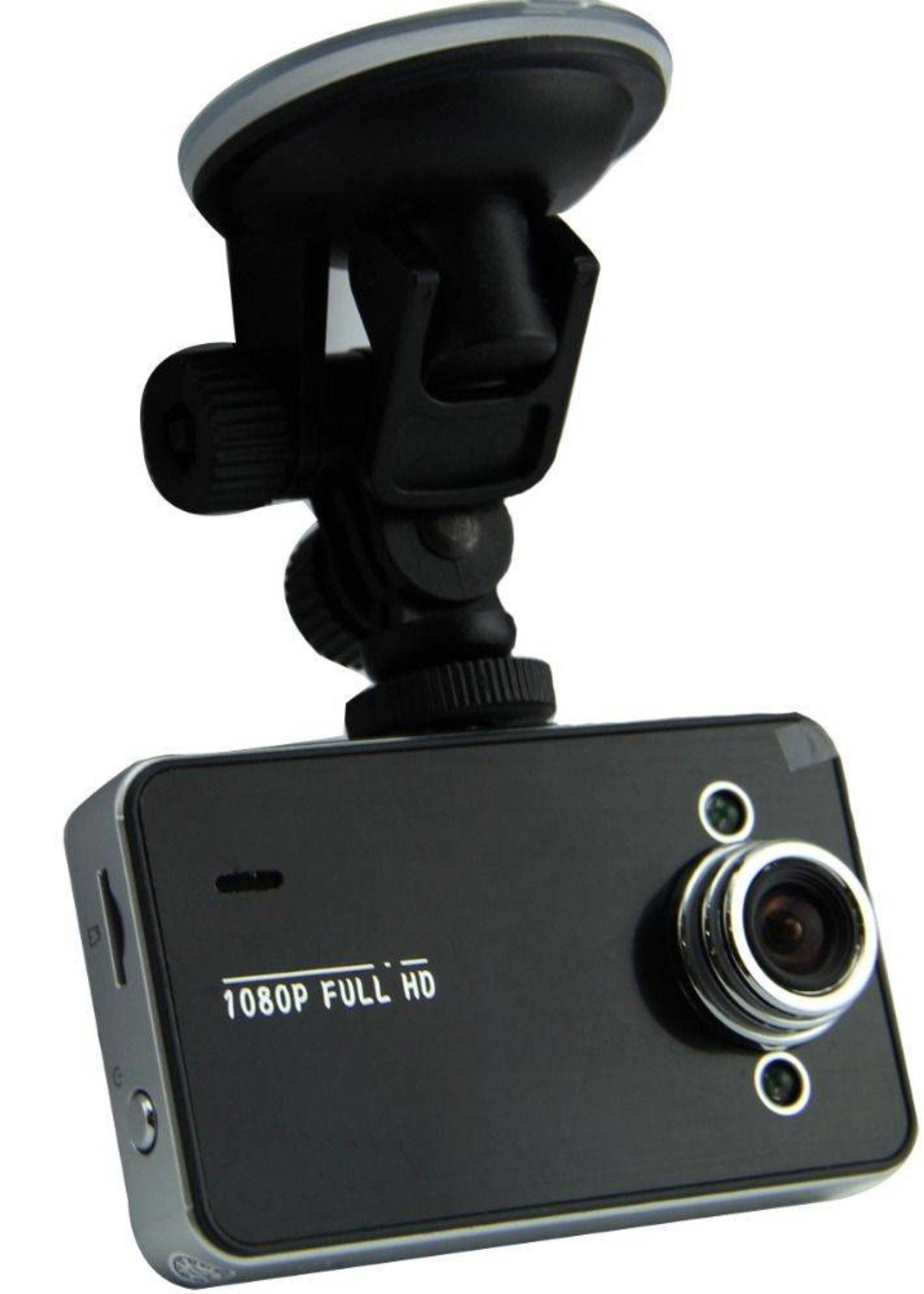The image features a sleek, black car dash cam resembling an iPhone. The camera is rectangular with rounded edges and prominently displays "1080p FULL HD" in white text on the left side of the front panel. The right side features a silver, chrome-like circular lens with a zoom function, framed by screws above and below. The device is mounted via a black plastic stand and an adjustable arm. This arm connects to a black portion at the top of the camera, which includes a transparent circular suction pad for attaching to a car windshield. Additional features include a rectangular slot for an SD card on the upper left and a protruding circular silver button on the side. The camera's design includes a twisting plastic attachment ensuring it can be adjusted to various recording angles. Two smaller lenses are also present, one above and one below the primary lens, enhancing its functionality. The entire outline of the camera is accentuated with a silver plastic trim, completing its modern aesthetic.